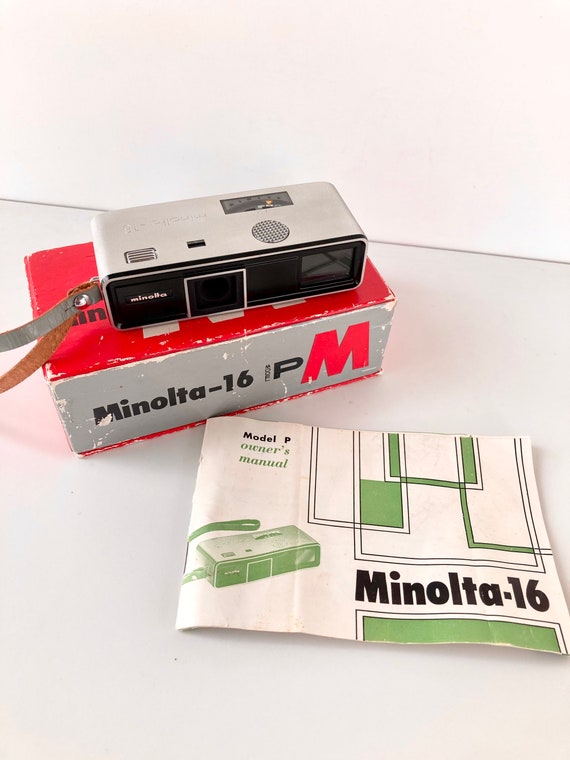This is a detailed photograph showcasing a vintage Minolta 16P camera set on a weathered, red and grey box, likely for sale on eBay. The box, with a red top and grey sides, clearly displays "Minolta-16" text in black and features a distinct red "M" on the side. The analog camera itself is an old-fashioned model, characterized by its grey and black color scheme, with "Minolta" inscribed in grey text next to the lens on its black front. The camera, approximately four inches long, three inches wide, and one inch tall, includes a dial on the top right and a wrist strap, indicating its vintage design. Beside the box rests a worn Minolta 16 owner's manual, notable for its rippled off-white cover and green box design elements. The manual prominently displays "Minolta 16" in bold black letters and features an angled image of the camera itself on its cover, with additional text reading "Model P Owner's Manual" at the top right. The entire arrangement is set on a white table top, capturing the nostalgic essence of this classic photographic equipment.